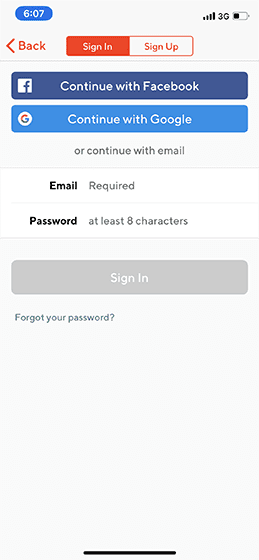Screenshot Description: 

The image showcases a detailed screenshot of a cell phone's interface. The top of the screen features an off-white background transitioning into a white background at the bottom. Prominent in the upper section is a blue rectangular oval shape with white lettering that displays the current time as 6:07. In the upper right corner, black icons depict four Wi-Fi bars, a 3G connection, and a battery level at approximately 33%.

To the upper left, there is an orange back arrow accompanied by the word "Back" also in orange. At the center top, two buttons are visible. The left button is solid orange with white lettering stating "Sign in," while the right button is solid white with orange lettering labeled "Sign up."

Beneath these buttons lies a light gray separating line followed by dark blue rectangular bars. The first bar on the left contains a Facebook icon, and in the center, white text reads "Continue with Facebook." Below this bar is a lighter, almost turquoise blue rectangular section featuring a white circle with the multicolored Google "G" icon on the left, accompanied by white text that reads "Continue with Google."

Further down, the screen shows the option "or continue with email" just above another gray separating line. Subsequent sections delineate fields for email and password input. The email field is labeled in bold black text "Email" with "Required" in light gray text. The password field is marked with "Password" in dark black text and a note on the right in gray stating "At least eight characters." Another gray line separates these input fields from a long rectangular gray bar that bears white text reading "Sign in."

At the very bottom left corner, in dark gray text, the phrase "Forgot your password?" is displayed, providing an option for password recovery.